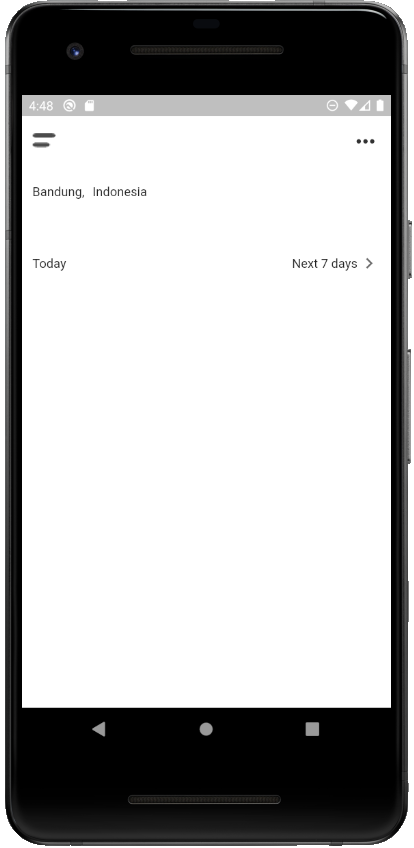This image depicts a smartphone screen with meticulously detailed elements. The phone itself has black borders at the top and bottom. At the bottom center, there's a horizontal gray bar. Starting from the top left of the screen, the time is displayed as "4:48," and on the top right, both the battery and Wi-Fi icons are neatly positioned.

Just below this, slightly on the left, there are two very small lines followed by three small dots. Below these icons, the location is shown, reading "Bandung, Indonesia." Directly beneath this, on the left side, is the word "Today," while on the right-hand side, it states "Next 7 days" accompanied by an arrow. All this text is rendered in black against a backdrop that transitions from gray at the very top to a predominantly white background.

At the bottom of the screen, three gray icons are visible: a sideways triangle on the left, a circle in the middle, and a square on the right. A subtle gray borderline outlines the left and right edges of the smartphone screen, framing the image completely.